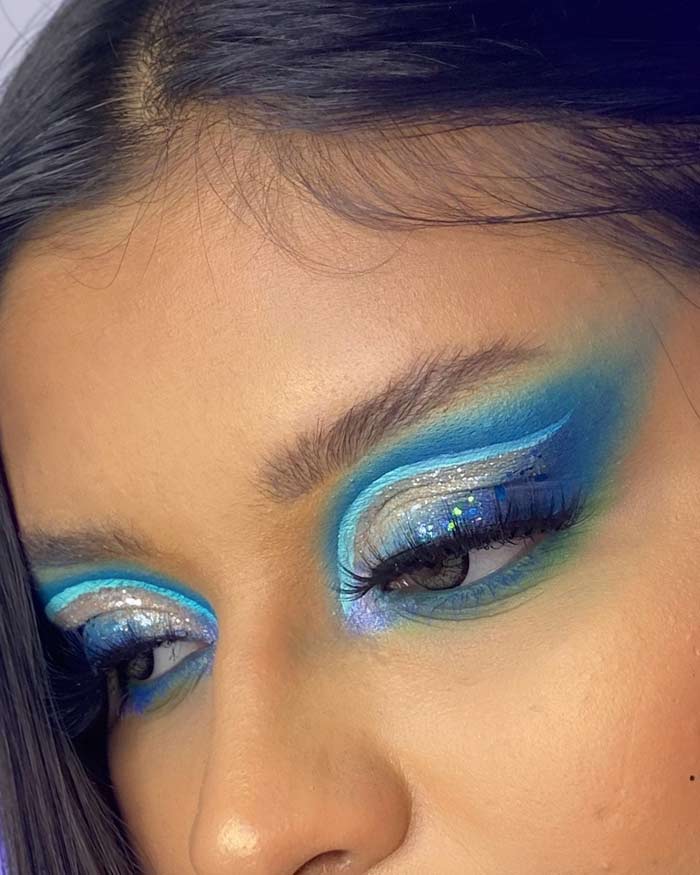The image is a very close-up, color photograph of a young woman's eyes and the upper part of her face. Her face is slightly tilted down and to the left, with her eyes half-open and looking in the same direction. She has dark brown or black hair peeking into the frame, and her tan skin is complemented by a heavy application of makeup. Her eyebrows are thin, and she is wearing elaborate, colorful eyeshadow. The eyeshadow features a medium blue base with a light blue swish line extending from the corner to the outer edge of her eyes. A sparkly silver line accentuates the contour of her eye, and a shimmery blue color highlights the top of her eyelid. The lower eyelid is adorned with medium green eyeshadow that has hints of blue, which doesn't extend far. She has long, thick black eyelashes that suggest extensions, and her makeup overall has a glittery, futuristic appearance. The partial view of her cheek, most of her nose, and a bit of the top of her head reveals a youthful, possibly teenage girl's visage that exudes beauty and meticulous detail in her makeup application.